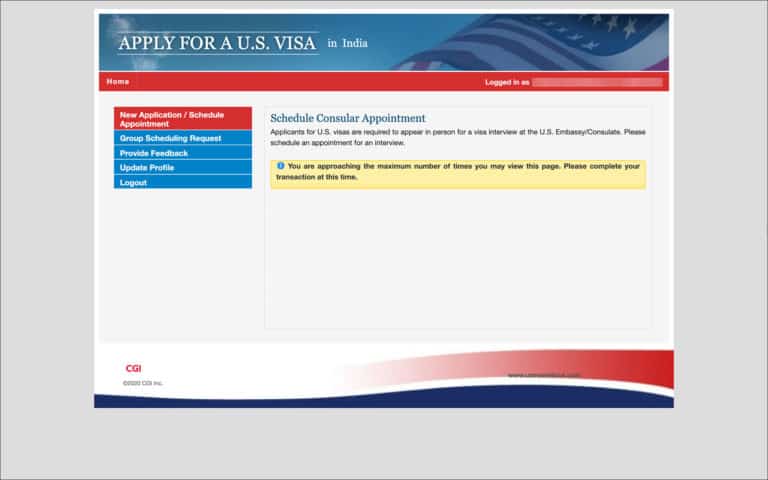Screenshot of a Web Page for U.S. Visa Application in India

The image captures a web page set within a gray background. Dominating the top portion of the screen is a blue banner with an American flag waving in the wind positioned at the far right. On the left side of the banner, it reads, "Apply for a U.S. Visa in India."

Directly below this is a red notification bar displaying the text: "Name, Logged in as," followed by an area that has been intentionally blurred out for privacy.

A vertical menu is located on the left side of the screen, listing the following options:
- "New Application/Schedule Appointment" (highlighted to indicate it has been selected),
- "Group Scheduling Request,"
- "Provide Feedback,"
- "Update Profile,"
- "Log Out."

The main section on the right side of the page is headed with "Schedule Consular Appointment," accompanied by text explaining that applicants for U.S. visas must attend an in-person interview at a U.S. Embassy or Consulate, and prompting users to schedule their appointment.

Just below this section is a yellow text box warning users, stating: "You are approaching the maximum number of times you may view this page. Please complete your transaction at this time."

The bottom of the screen is accented with a wavy blue and red design. In the bottom-left corner, the logo "CGI" is displayed. 

Notably, the screenshot does not include any images of people, animals, plants, flowers, or trees.